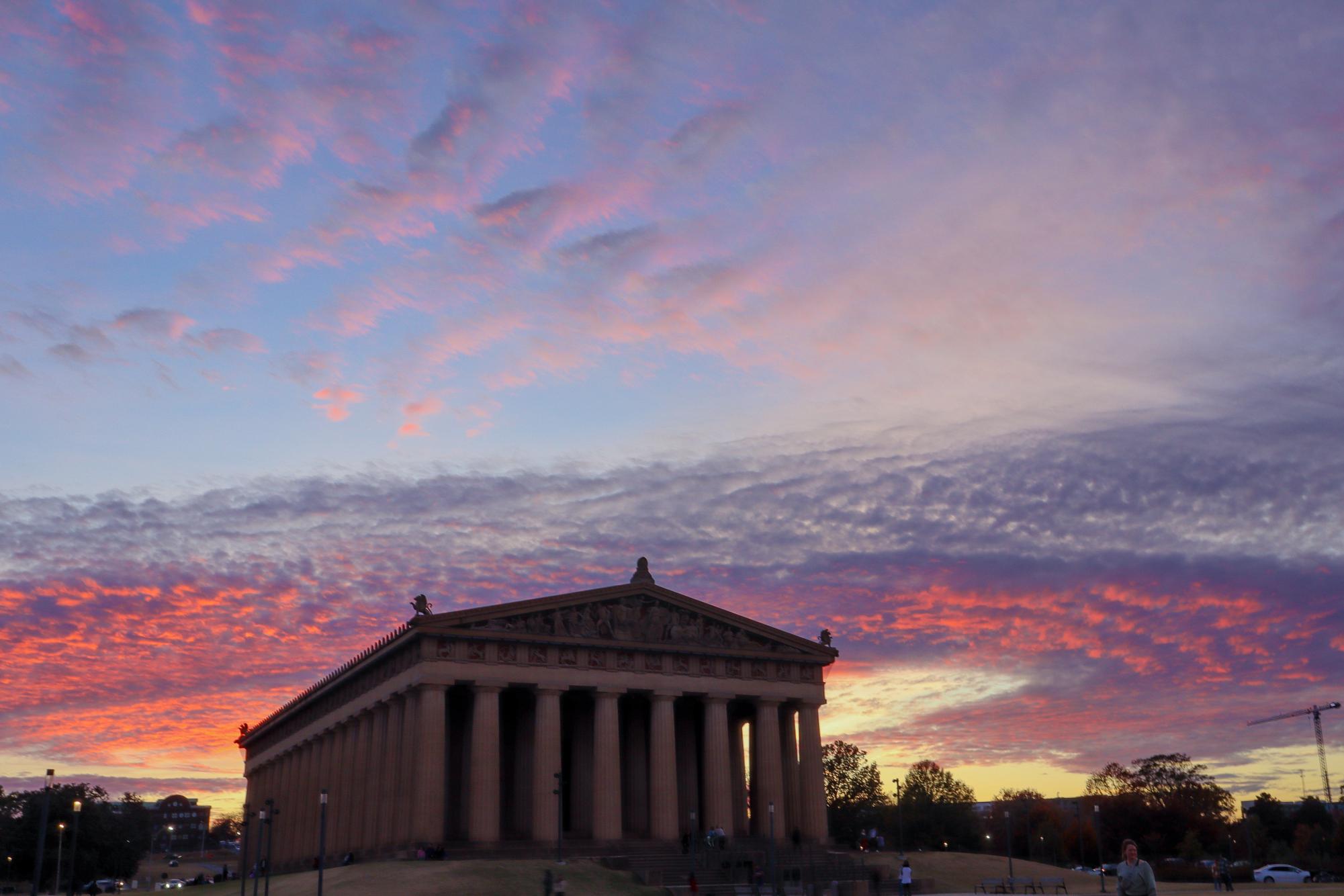In this evocative image, a replica of the Parthenon is captured in an American city, possibly Nashville, Tennessee. The majestic stone building, adorned with numerous columns, sits within an urban environment, evidenced by the presence of light poles, American cars, and a few distant individuals. In the bottom right corner, a small white car is visible. Trees, sparse with leaves, border the image on the right side. The real spectacle, however, is the mesmerizing sky at sunset dominating the scene. The sky transitions from a base of soft white at the horizon to a stunning palette of pinks, oranges, purples, and deep blues. Billowy pink clouds are scattered across the top, creating a dynamic contrast against the darker hues, while a rim of vibrant orangey-pink and yellows near the skyline suggests the sun has just set behind the Parthenon, casting the whole scene in a surreal, enchanting glow.